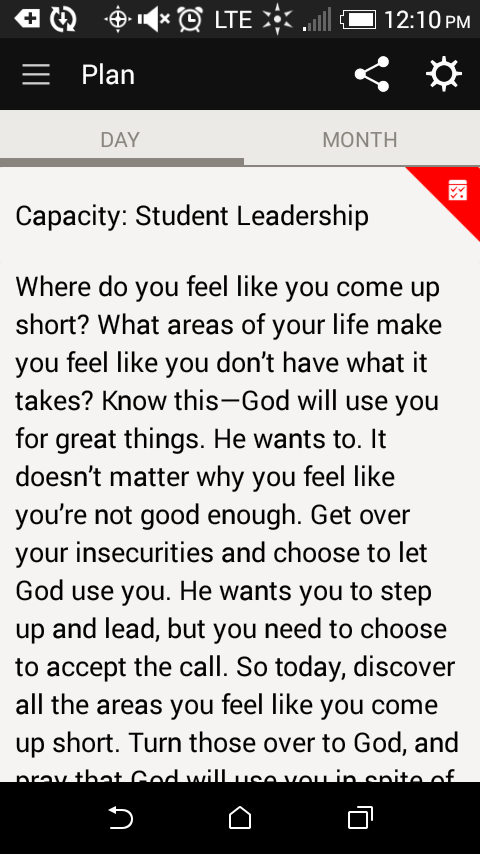The image depicts a screenshot from a mobile device, likely an Android phone, indicated by the presence of standard widgets and icons such as battery level, time, and sharing options on the top banner. The content appears to come from a planning or motivational app, with a layout highlighting the day and month. The visible text on the screenshot reads, "Capacity Student Leadership. Where do you feel like you've come up short? What areas of your life make you feel like you don't have what it takes? Know this, God will use you for great things. He wants to. It doesn't matter why you feel like you're not good enough. Get over your insecurities and choose to let God use you. He wants you to step up and lead, but you need to choose to accept the call. So today, discover all the areas you feel like you've come up short. Turn those over to God," though the last line is cut off. The entire message is presented in black and white, adding a stark, straightforward visual style to the already direct and motivational tone of the text.